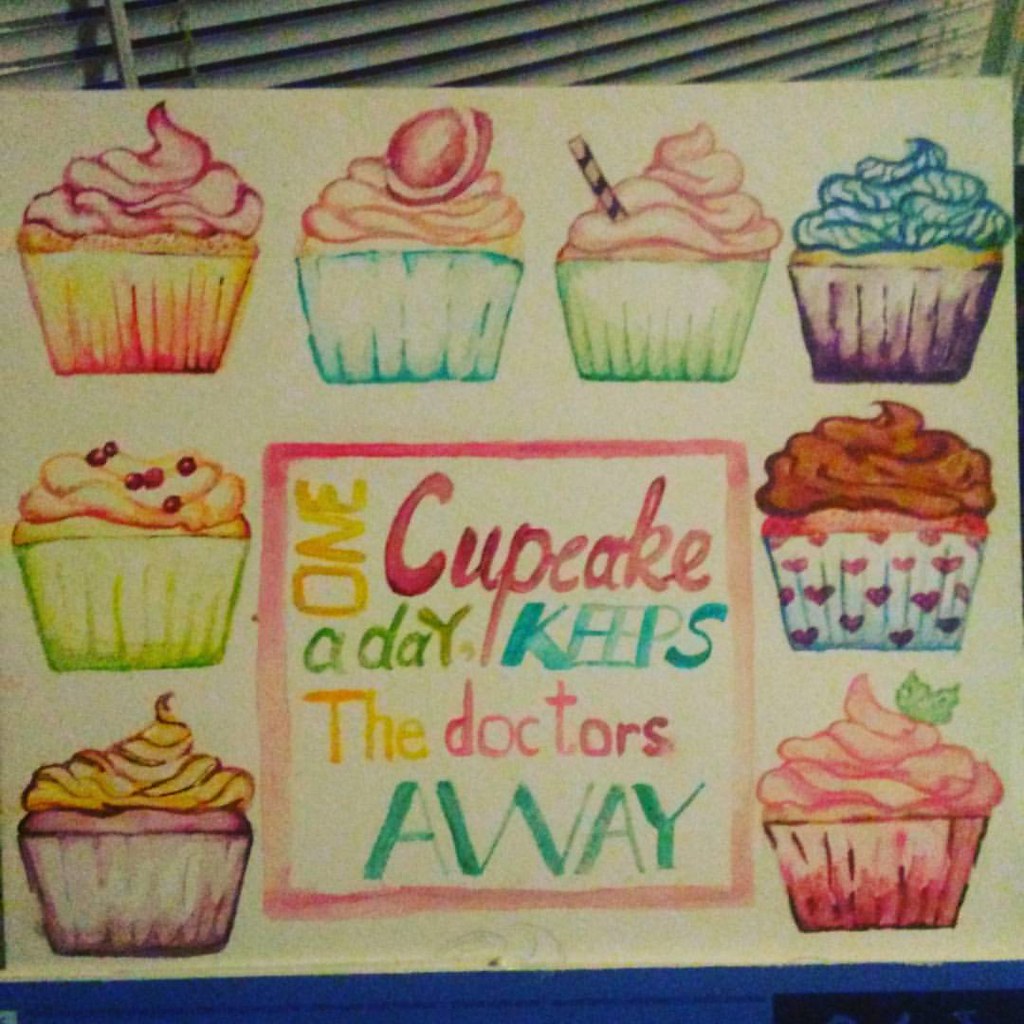The illustration is a detailed and vibrant mixed media artwork featuring eight uniquely decorated cupcakes arranged along the left, upper, and right sides of a white paper background. Each cupcake is distinct, showing an array of colorful frosting and varied wrappers: a pink wrapper with pink frosting topped with a green leaf, a white wrapper with hearts and brown frosting, a purple wrapper with blue frosting, a green wrapper with pink frosting adorned with candy, a blue wrapper with yellow frosting and a football decoration, a yellow wrapper with pink frosting, a green wrapper with yellow frosting and red dots, and a purplish wrapper with yellow frosting. The center of the paper features a pink square enclosing text in various orientations and colors—yellow, red, green, and blue—declaring, "One cupcake a day keeps the doctor away." The illustration is propped against a window with partially opened louvered plastic blinds. Although the image captures the artistic skill and vibrant charm of the cupcakes, it was taken with an amateurish quality.